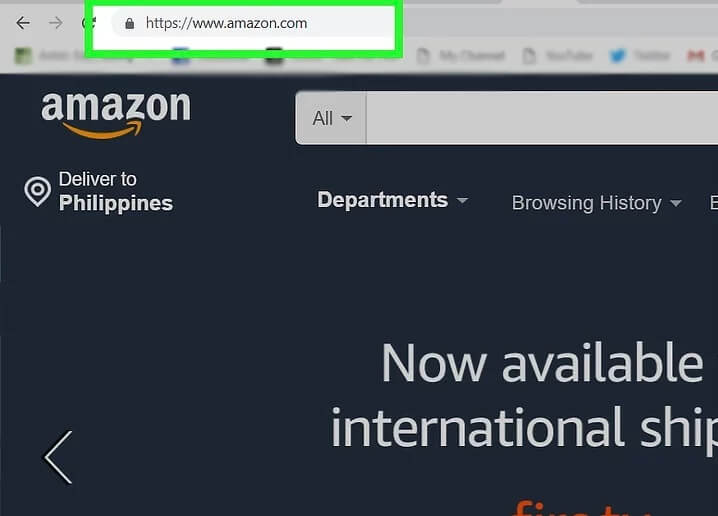A screenshot taken from a Safari browser, featuring the upper left section of the Amazon.com webpage. The screenshot highlights the URL area, enclosed by a neon green outline around the URL bar, indicating https://www.amazon.com with a secure padlock icon. The webpage's header showcases a navy blue background. The Amazon logo is prominently displayed on the left, while a location pointer icon is situated nearby, with "Deliver to Philippines" written in white text. Only a cropped view focusing on this section of the webpage is visible, excluding the rest of the content.